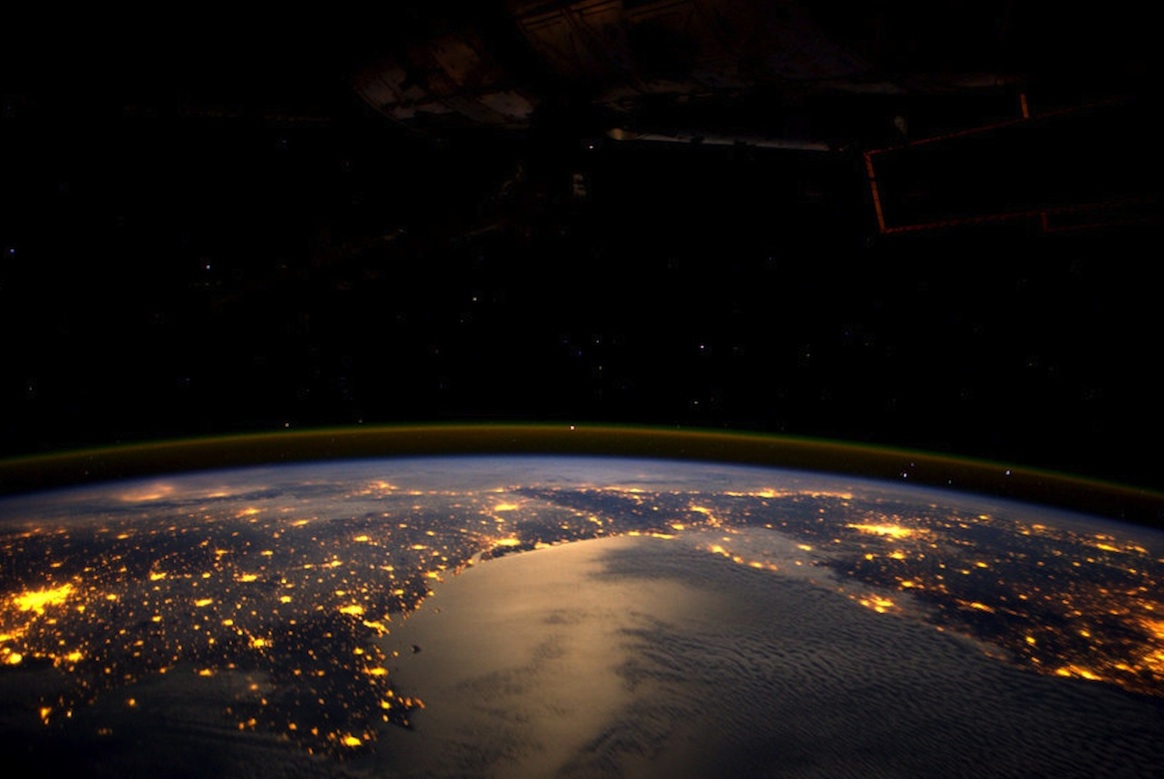This captivating aerial photo, likely taken from space, showcases a detailed view of Earth at night. Dominating the scene are several continents illuminated with golden-hued lights that intricately outline the landmasses, creating a breathtaking visual of interconnected regions. Europe seems prominent in this view, its boundaries clearly visible amidst the darkness. The serene expanse of water, rendered in whitish-blue, accentuates the land, adding depth to the scene. Above, the pitch-black sky is dotted with tiny white stars, enhancing the surreal nature of the image. A faint silhouette of a device also hovers, hinting at the high vantage point from which this remarkable photo was captured.